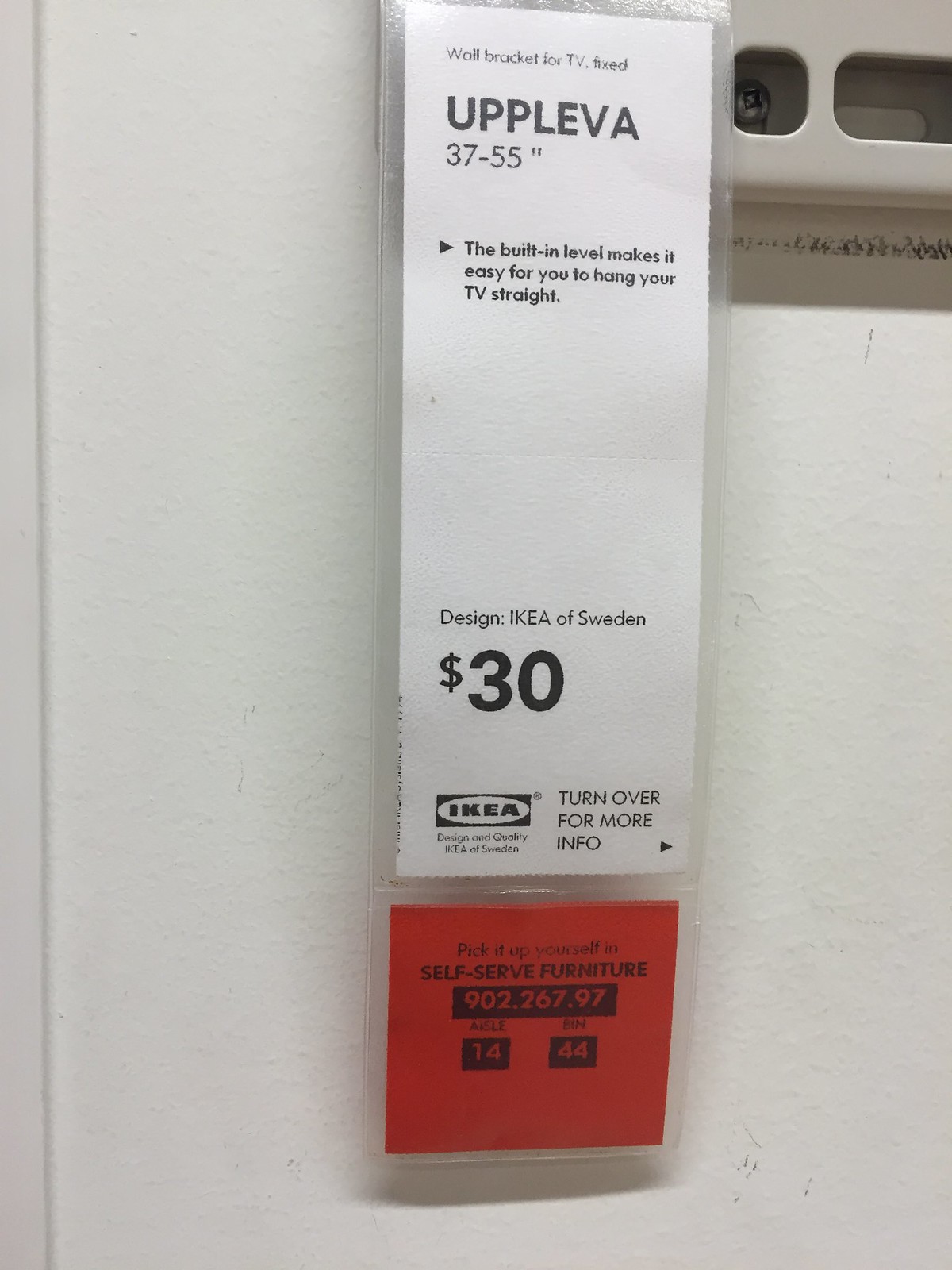The image captures an IKEA price tag sign displayed against a light khaki background, presumably mounted on a tan-colored metal bracket. The sign, encased in a clear plastic covering, prominently features a white label at the top and a red tab at the bottom. The top portion of the label, resembling a bookmark shape, reads "Wall Bracket for TV Fixed," accommodating TVs ranging from 37 to 55 inches. Below this, in block capitals, it states "UPPLEVA," followed by a description in smaller text: "The built-in level makes it easy for you to hang your TV straight." Further down, it notes "Design and Quality IKEA of Sweden," accompanied by the IKEA logo. The price of the bracket is clearly marked as $30. Towards the lower segment of the white label, there is an instruction to "Turn over for more info."

The bottom red section of the tag provides additional directives, stating "Pick it up yourself in self-serve furniture" and includes a specific code, "902.267.97," for locating the item. This section also features small black text with unreadable words and two black squares with the numbers "14" and "44" inscribed in red. 

The entire setup is mounted against a simple white wall, highlighting the clear, practical design of the sign that adheres to IKEA's functional and user-friendly aesthetic.